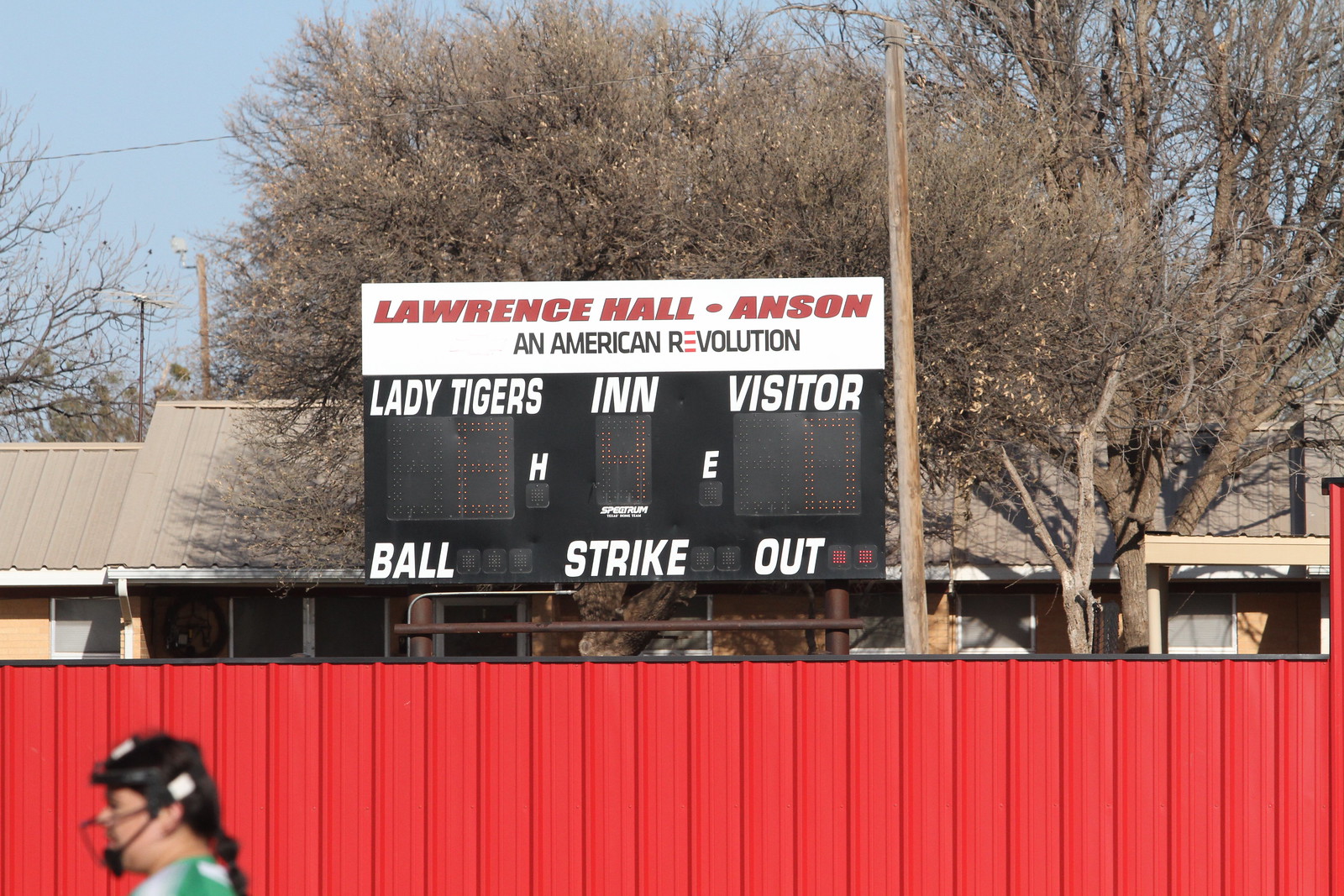This photograph captures the detailed scene at an outdoor baseball stadium. Dominating the center is a rectangular scoreboard. At the very top, against a white background, bold red text reads "Lawrence Hall, Anson." Below it, smaller black text declares "An American Revolution," with the 'E' ingeniously stylized as three red horizontal lines. The middle section of the scoreboard, set against a black background, displays the home team name "Lady Tigers" on the left, the inning 'N' in the center, and "Visitor" on the right. The scoreboard shows that the Lady Tigers have scored 8 runs, the inning is in the 4th, and the Visitors have yet to score. Below, indicators for Ball, Strike, and Out are present; with no balls, no strikes, and two outs currently recorded.

In the immediate surroundings, a light brown utility pole rises just to the right behind the scoreboard, adorned with electrical cords. Background scenery includes rooftops of several houses, whose light brown color blends with the seasonally leafless or brown-leafed trees. The setting is bathed in a clear blue sky, suggesting a cloudless day.

In the foreground, a bright red tin fence stretches across the scene. At the bottom left corner of the image, partially cropped, a softball player stands out. Her headgear, face mask, and black-ponytailed hair are visible, and she seems to be watching attentively to the left while donning a green jersey. The overall impression hints at the calm yet focused atmosphere of a game in progress.